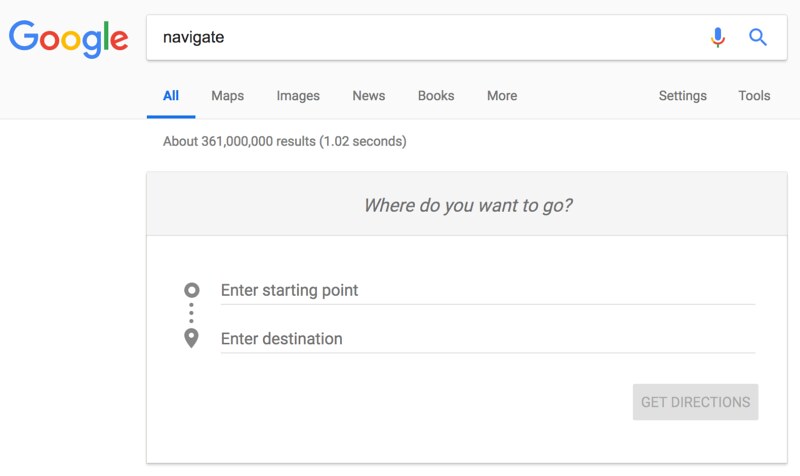The image showcases a Google search page. At the top, the iconic Google logo is prominently displayed, followed by the search bar with the word "navigate" typed in black letters. On the right side of the search bar, the microphone button and magnifying glass icon are visible. Beneath the search bar, the word "All" is highlighted in blue, accompanied by other options such as Maps, Images, News, Blogs, More, Settings, and Tools. The search results indicate approximately 361 million results found in 1.02 seconds. Below this, a gray section prompts, "Where do you want to go?" and features text fields labeled "Enter starting point" and "Enter destination," connected by a circular route icon. At the bottom right, a gray tab labeled "Get directions" is visible.